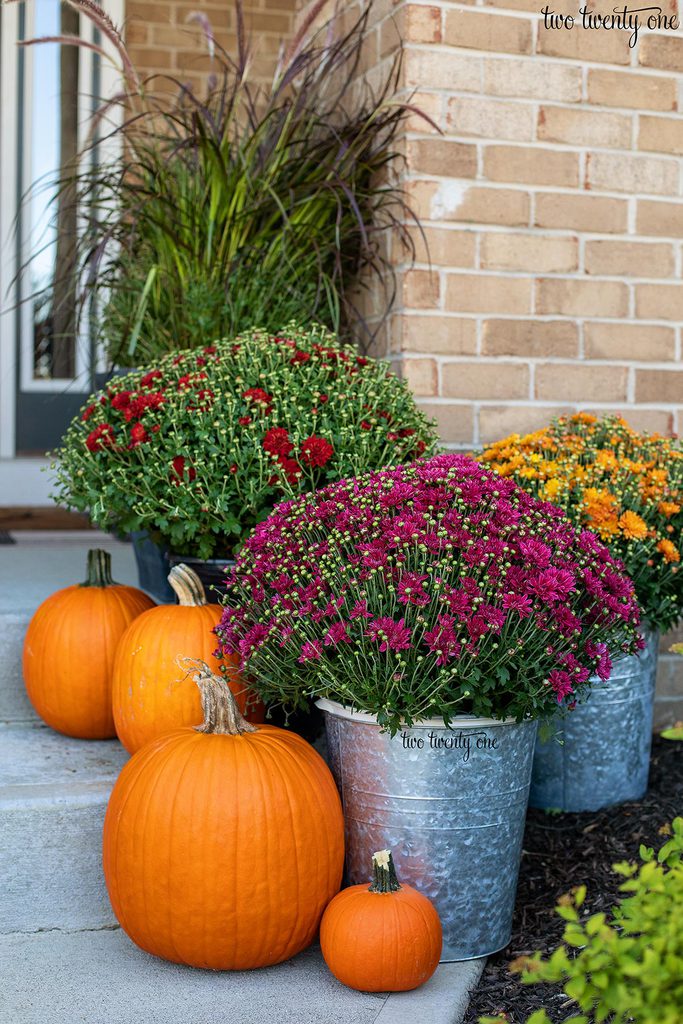This captivating photograph, watermarked “221,” showcases the meticulously arranged front steps of a brick residence. Dominating the scene are three chic galvanized buckets, each brimming with a vibrant array of flowers. The top step features a metal bucket with tightly packed red blooms, complemented by a second bucket on the lower step filled with magenta flowers. Nestled to the right, an additional bucket contains a striking mix of orange and yellow flowers. At the farthest edge, delicate fern-like greenery adds a whimsical touch. 

Sharing the spotlight are four uncarved pumpkins, strategically positioned across the two concrete steps: two medium-sized pumpkins grace the lower step, while the larger pumpkin stands on the cement ground beside a tiniest one. The brick backdrop, a harmonious blend of tan and brown hues, further enhances the visual appeal.

Adjacent to this welcoming arrangement lies a tidy flower garden, marked by a bed of mulch beneath the buckets. The overall display is both aesthetically pleasing and thoughtfully curated, capturing the essence of an inviting home entryway.